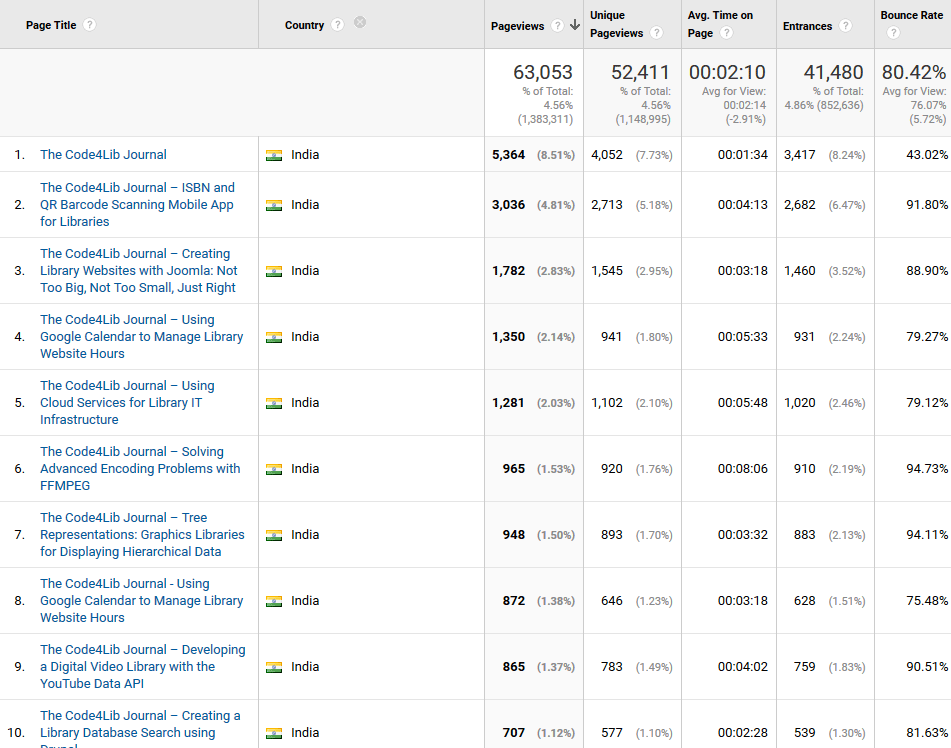A detailed chart showcases data in rows and columns. The chart consists of 7 columns and 11 rows. Each column header is displayed in bold black text, accompanied by a white circle with a gray question mark inside, positioned to the right of the text. The columns are of varying widths, with the first two being the largest.

The first column is titled "Page Title," and the second column is labeled "Country." The remaining columns include various metrics such as page views, which features a gray downward arrow to the right of the question mark symbol.

Observations about the data in the rows:

1. The first row is devoid of values in the "Page Title" and "Country" columns, but it includes numerical data and percentages in black text for the remaining columns.

2. The next 10 rows contain:
   - "Page Title" values in blue text in the first column.
   - The second column consistently displays the flag of India followed by the text "India."
   - The remaining columns contain data in black text, with occasional gray text in parentheses to denote additional information.

The arrangement of colors and symbols within the chart aids in differentiating between various types of data and their significance.